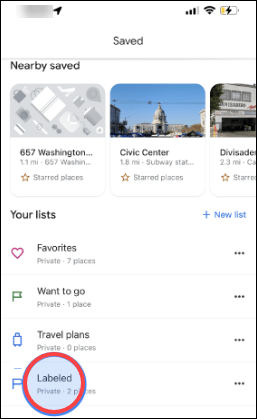A cell phone screenshot displaying an interface has been shared, with some elements obscured for privacy. At the top of the screen, several icons are partially blurred out, leaving a rectangular blur that conceals specific details. The battery icon indicates it is charging and was previously low.

The screenshot shows a section titled "Nearby Saved," with three rounded rectangle boxes underneath. One of these boxes reveals "657 Washington Civic Center," but the remainder of the text is cut off. Below this are options labeled "Your List" and "Plus New List." Underneath that, there are sections for "Favorites," "Want to go" marked with a green flag, "Travel plans" accompanied by small luggage icons, and a "Labeled" section.

In the "Labeled" section, which is marked as private and contains two places, a blue highlight is visible. Additionally, a digitally added red circle emphasizes this area. The overall image captures someone's organized and personalized list on their device, with specific visual highlights and tasks indicated.